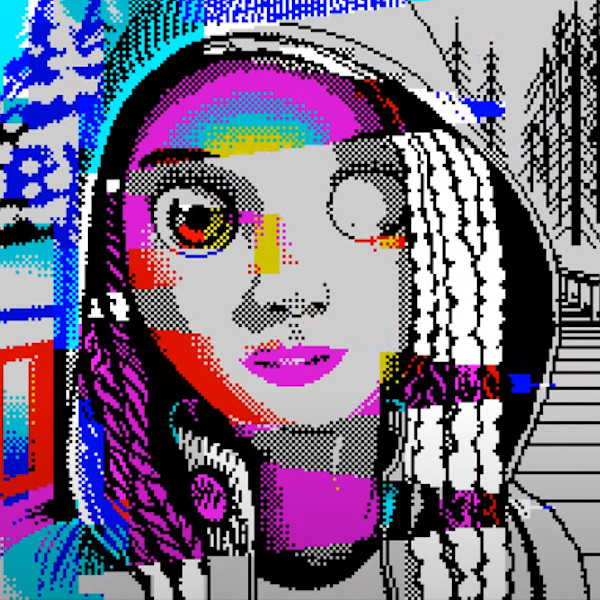This digital artwork depicts a stylized, pixelated image of a girl with a hood, created using older computer technology. The piece features a mix of abstract elements with a wide range of colors—grayscale, vivid purples, blues, reds, and yellows. The girl's long hair falls on both sides of her face, which is mostly gray and pixelated. Her left eye is colorful with red and yellow tones, while her right eye is an empty circle. She has distinctive purple lips and stands in the foreground, giving the impression of being close to an imagined camera. The background portrays a natural setting with a bridge or sidewalk and trees. On the right, the trees are uncolored outlines, while on the left, they are covered in snow and appear blue. The contrast between colored and grayscale elements creates an intriguing, abstract scene.